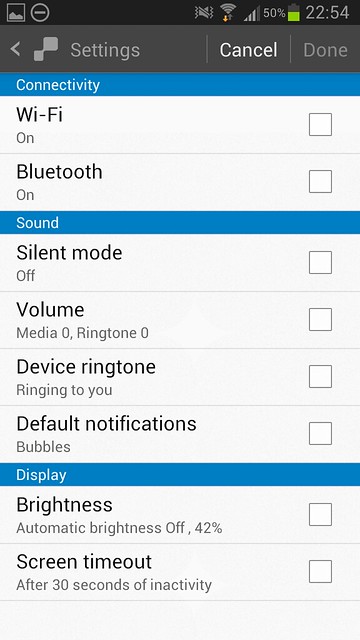This is a detailed cell phone screenshot featuring various interface elements and settings. At the very top, there is a thin black bar where the information is displayed in gray. On the upper left corner of this bar, there is a photograph icon followed by a notification symbol indicating that notifications are turned off. Further to the right, the sound icon is also turned off. The Wi-Fi signal shows three bars with an orange downward arrow beneath it, indicating network activity or status. To the right, the battery level is about 60% with the battery icon partially filled with green, and the current time displayed is 22:54.

Below this top bar, there is a wider gray section. On the left side of this section, there is a gray back arrow, a gray speech bubble, and to its right, the word "Settings" in gray font. On the right-hand side of this section, there are three textual elements: "Cancel" in bold white, and "Done" in gray on the extreme right.

Beneath this gray section, there is a turquoise blue divider with the word "Connectivity" written in white on the left side. Below this, there are two white sections: the first labeled "Wi-Fi," which is turned on, but its checkbox on the right is not checked. The second section is labeled "Bluetooth," which is also turned on, with its checkbox similarly unchecked.

Following this, there is another turquoise blue divider labeled "Sound" in white on the left-hand side. Under this section, several options are listed, each with an unchecked checkbox on the right: "Silent mode" (which is off), "Volume," "Device ringtone," and "Default notifications."

Finally, another turquoise blue divider that says "Display" in white on the left leads to two more lines with checkboxes on the right-hand side, both unchecked. The left side of these sections is labeled with bold black lettering reading "Brightness" and "Screen timeout."